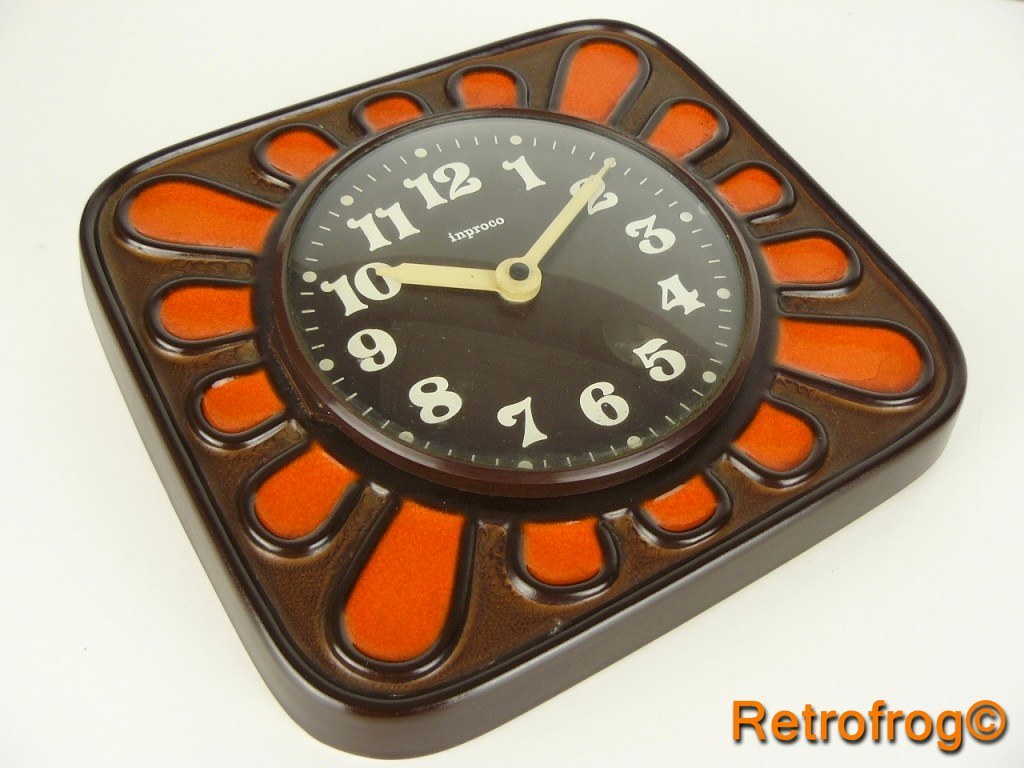This image depicts a top-down view of a square-shaped clock with intricate details and vibrant colors. The clock features light gray outer edges, but only the left and bottom sides are visible, as the right and top edges fall outside the frame. The clock's border is brown, creating a warm contrast to its inner elements. Surrounding the clock face, there is a series of bright orange shapes resembling the tips of fingers, adding a unique and playful design element.

Positioned at the bottom right of the image is orange text that reads "Retrofrog," accompanied by a small circled "C" emblem to the right of the "G." The clock face showcases numbers from 12 to 12 in a circular arrangement, all rendered in white. The clock hands are tan-colored, with the short hand pointing at the 10 and the long hand at the 2, indicating the time. This visually striking image combines retro design elements with a modern touch, making it both functional and aesthetically appealing.